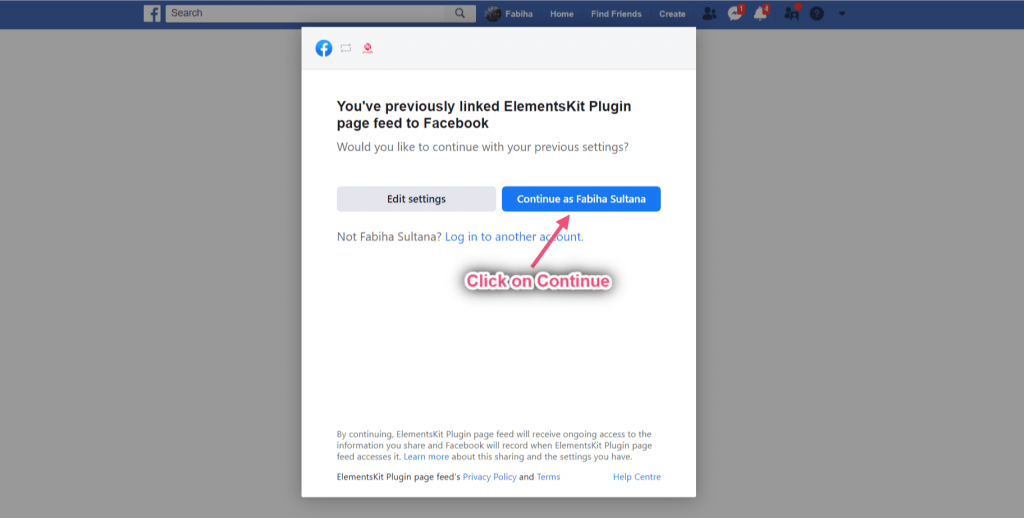This screenshot depicts a Facebook interface with a prominent pop-up dialogue box overlaying the main page. In the center of the screen, a large white box dominates the view. In the top left corner of this box, the recognizable blue circle featuring a white 'F' logo representing Facebook is displayed.

Just below the logo, centered within the box, black text reads: "You've previously linked Element Kit plugin Element Kit plugin page feed to Facebook." Directly underneath, a prompt in light gray text asks: "Would you like to continue with your previous settings?"

Further down the box, two clickable options are presented. On the left, a gray button with black text in the center says "Edit Settings." On the right, a blue button with white text in the center reads: "Continue as Fabitha Sultana," indicating the account’s user name.

Highlighting the action to be taken, large red text with a white and black outline states "Click on continue," complemented by a red arrow pointing towards the blue "Continue" button.

In the darker background outside the pop-up, the faint layout of the Facebook site is visible, suggesting it is not the primary focus. The familiar blue horizontal navigation bar at the top includes the Facebook logo, a search box, and links to the user profile, home page, friend finder, Facebook Messenger, notifications, and other site pages.

Toward the bottom of the screen, small gray text mentions Facebook's ads and privacy policy, along with a blue link directing users to the Help Center, found in the very bottom right corner.